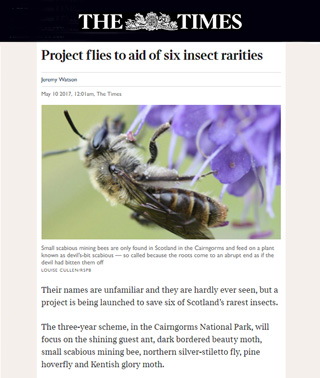**Detailed Caption:**

In this newspaper clipping from The Times dated May 10th, 2017, an article by Jeremy Watson and Louis Kolenabs announces the launch of a project dedicated to conserving six of Scotland's rarest insects. The article, titled "Project Flies to Eat of Six Insects Rarities," highlights the initiative centered in the Cairngorms National Park. One prominent image accompanying the text shows a Small Scabious Mining Bee resting on a flower, exemplifying one of the endangered species. These bees are exclusive to Scotland, where they thrive on the devil's-bit scabious plant, named so due to its roots appearing abruptly bitten off. The three-year conservation effort will also focus on the Shining Guest Ant, Dark Bordered Beauty Moth, Northern Silver Stiletto Fly, Pine Hoverfly, and the Kentish.